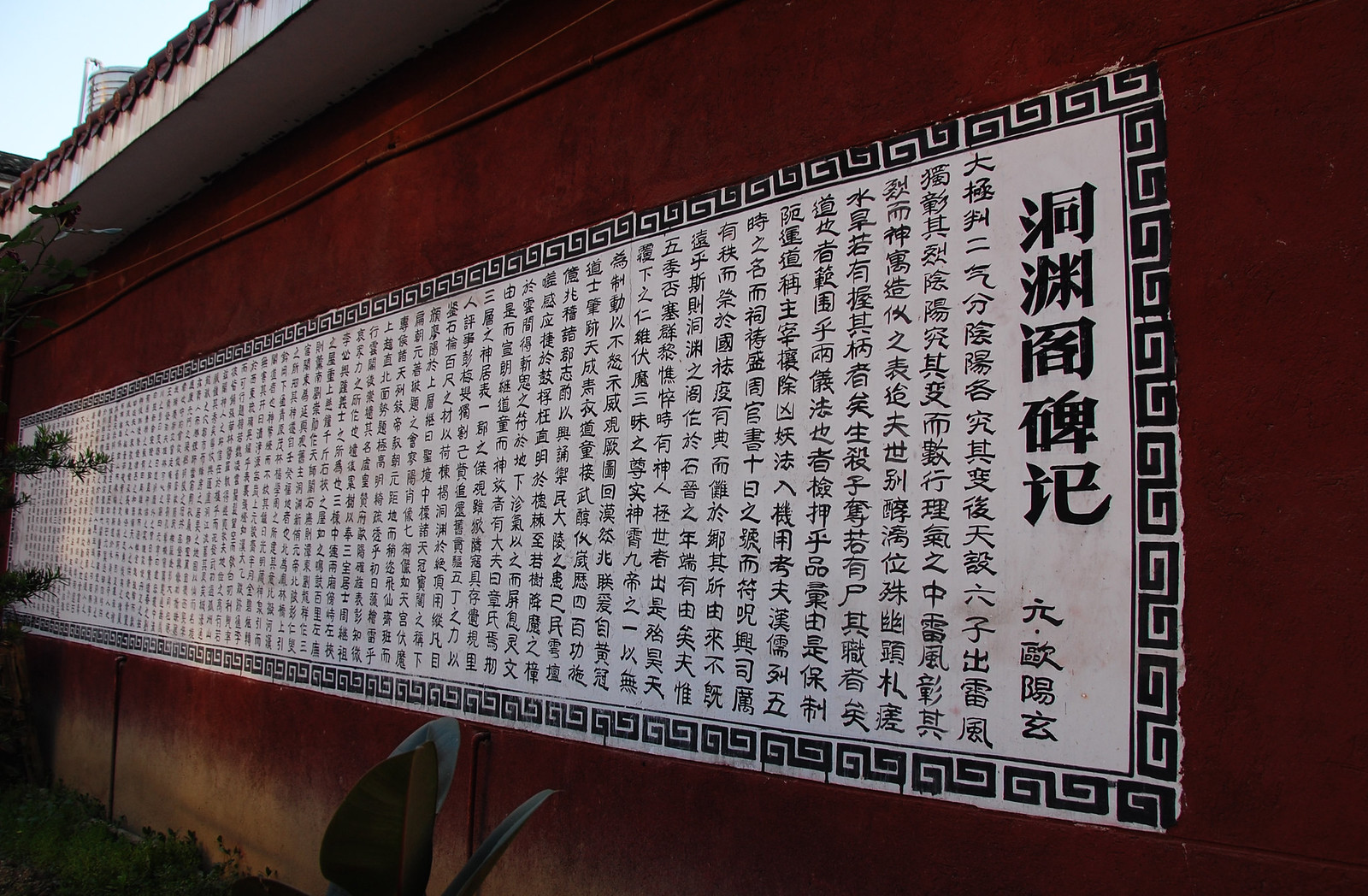The image depicts a long red-walled building in China, characterized by its dark red terracotta roofing. The focus is on a lengthy Chinese inscription set against a white background with a distinctive black-and-white square spiral border. This inscription runs horizontally along the upper part of the wall and includes larger Chinese characters positioned vertically near the right side. The area around the text is framed by intricate, alternating square spirals resembling a zigzagging tail. 

In front of this wall, a flower bed with broad green leaves and ivy starts to climb the inscription. The bottom of the wall appears brown and sandy, with dirt and some grass patches visible. The building's awning extends out above the wall, providing some shade. On the far left side of the image, branches and leaves of a tree intrude into the frame, while hints of blue sky and the edge of another tall building can be seen in the background, completing the scene with a touch of natural and urban blend.